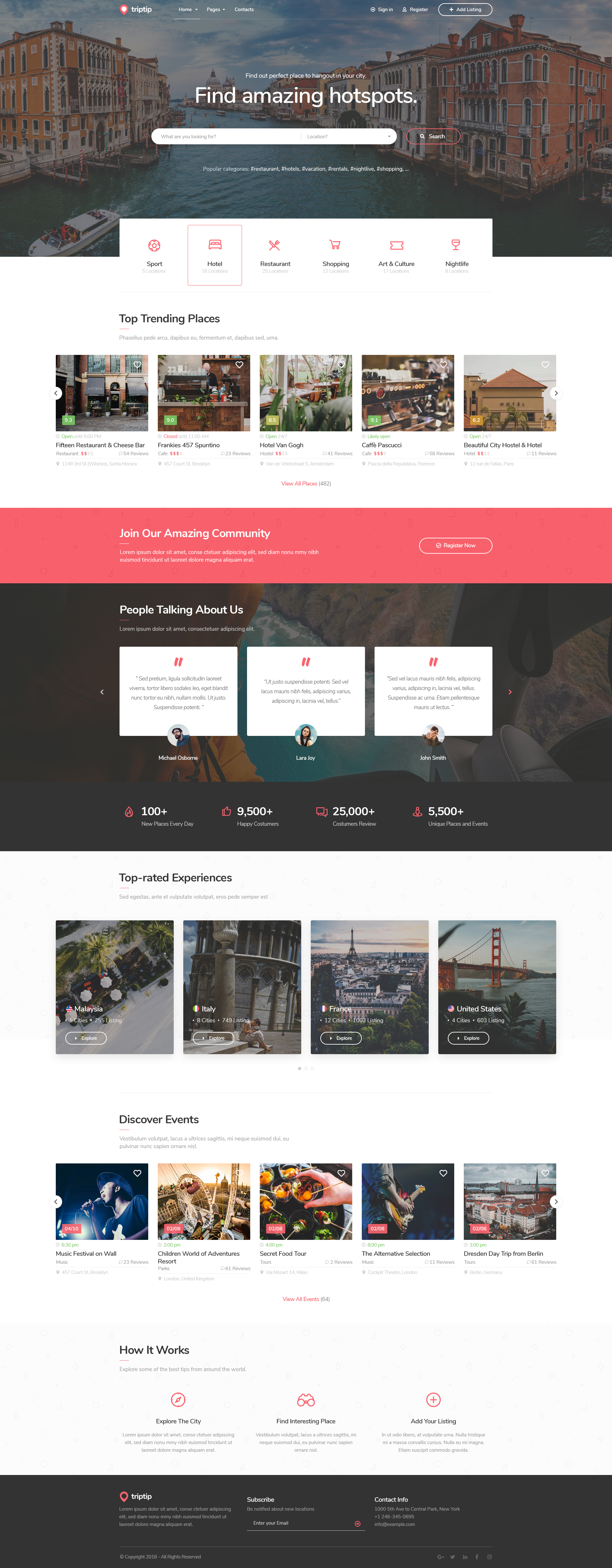This is a detailed screenshot of a visually appealing landing page. At the top, there's a hero image with a search bar designed to help users find amazing hotspots. Directly below, five options are displayed with accompanying icons for easy navigation. The next section is titled "Top Trending Places," showcasing five side-by-side images that highlight these destinations.

Following this, a prominent red bar catches the eye, featuring a button that highlights community contributions. Three detailed user reviews are presented beneath this section. An additional set of four images highlights other top-rated locations.

Further down, the page features "Discovering Events," with five side-by-side images illustrating various events. At the very bottom, the page provides a concise explanation of how the platform works, ensuring users have a clear understanding of its functionalities.